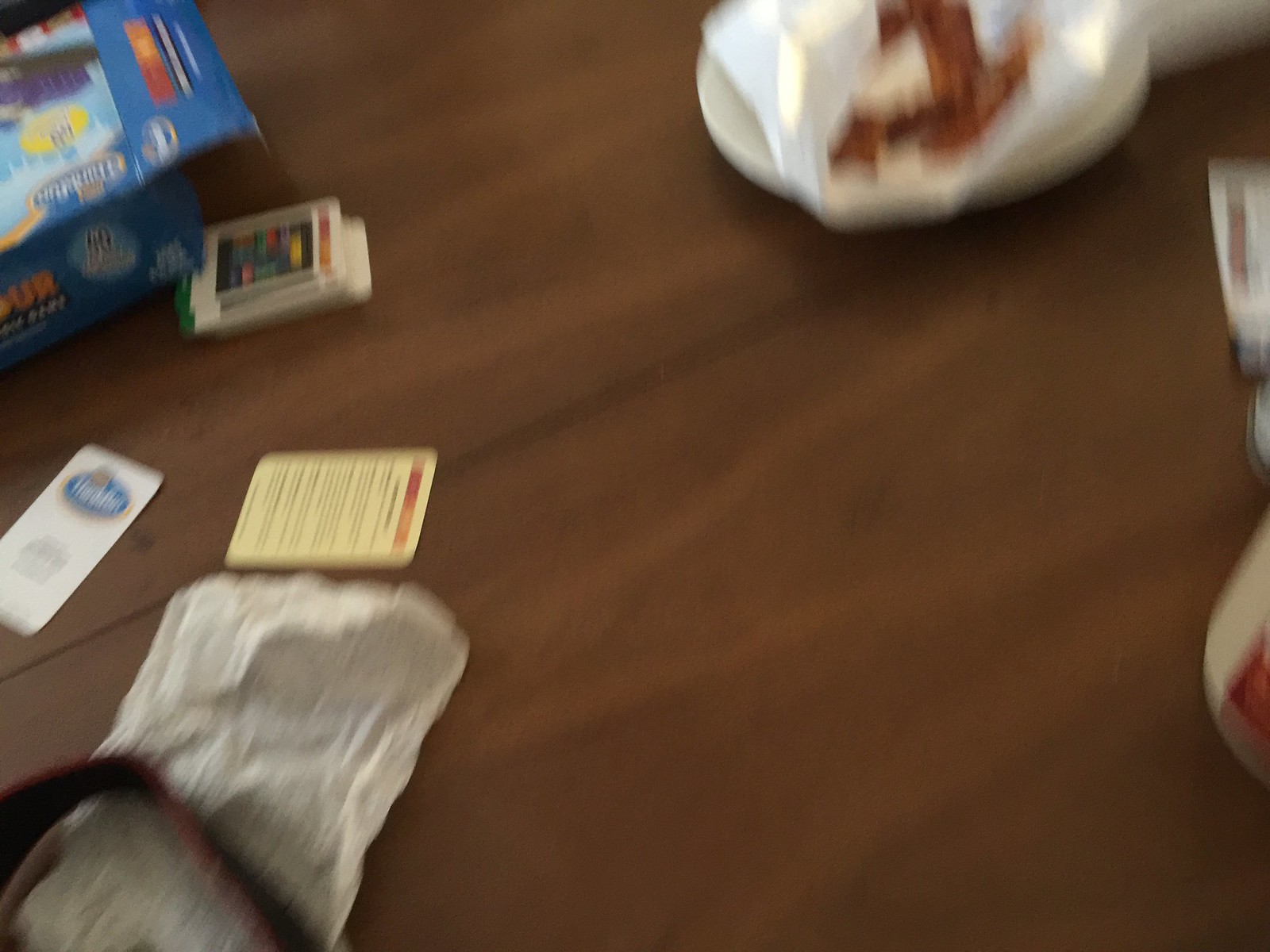A blurry photograph captures a wooden table with a noticeable grain pattern. On the table, there is a colorful box featuring blue, yellow, red, and several other colors, suggesting it is part of a game. Near the box lies a unique deck of cards intended for gameplay, distinct from a standard deck. A plate with indistinguishable contents sits near the cards, along with a spread-out napkin. The overall scene gives a casual and playful atmosphere, despite the lack of clarity in the image.